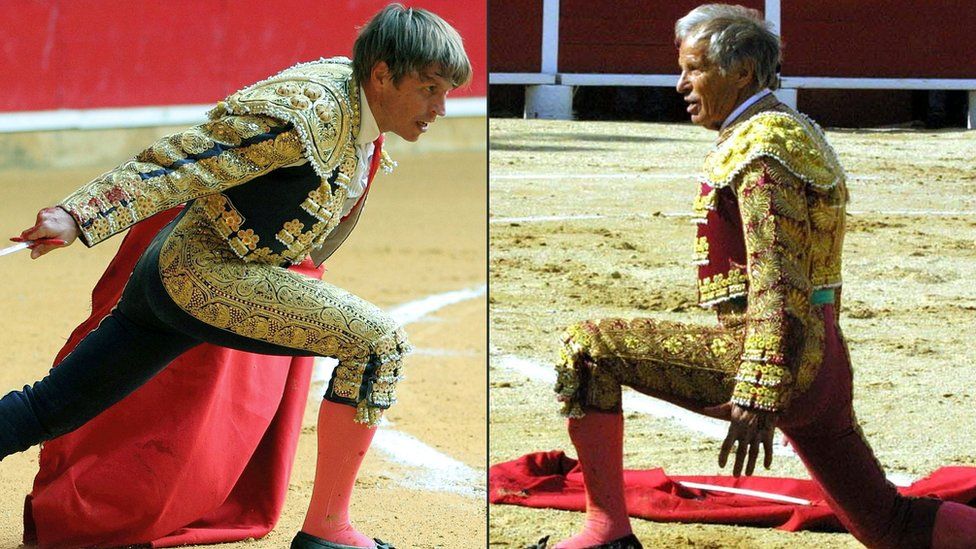This image is a composite of two separate photographs placed side by side, featuring two matadors each striking a powerful pose. The matador on the left is depicted leaning forward, as if about to kneel, dressed in an opulent black and gold suit adorned with intricate detailing on the shoulders, sleeves, and sides of the legs. He wears a white button-down shirt, red socks, black leather shoes, and a red tie under his elaborately decorated jacket. The matador's gray hair suggests a man of experience. Beside him, the matador on the right, who appears older with thinning gray hair, is captured in a genuflecting stance, his right knee touching the ground while his left knee forms a 90-degree angle. He is clad in an equally ornate red and gold suit, complete with similar decorations on the shoulders, sleeves, and the sides of his capri-style pants. His red cape lies dramatically on the ground next to him. Both men hold swords in hand, ready for the bullfight, with their vividly colored and richly embellished attire signaling their roles as seasoned bullfighters.